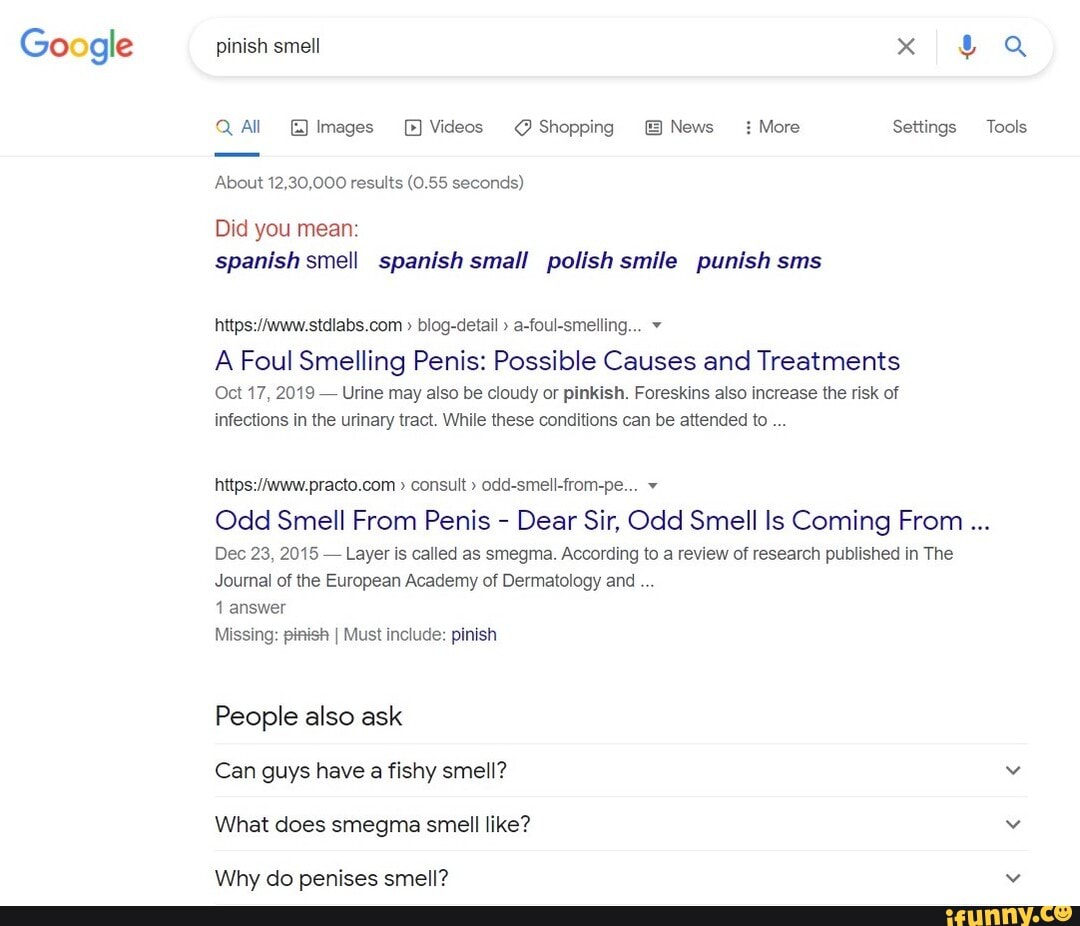This image captures a screenshot of Google search results, focusing on a search query that appears to be "finish smell" but was likely misspelled as "pnish smell." The search bar, positioned prominently at the top, displays a small "x" button for clearing the search term, a microphone icon for voice input, and a magnifying glass icon for initiating the search. Just above the search results is the top navigation menu, offering categories such as All, Images, Videos, Shopping, News, More, Settings, and Tools. 

The search results themselves include various suggestions and corrections like "Do you mean Spanish smell, Spanish small, Polish smile, Punish SMS." Below these suggestions are links to articles discussing topics related to penile odor, such as “foul smelling penis, possible cures and treatments,” “odd smell from penis, dear sir odd,” and an article titled "odd smell is coming from."

Additionally, there is a section labeled “People also ask,” featuring questions like “Can guys have a fishy smell?”, “What does smegma smell like?”, and “Why do penises smell?”. At the very bottom of the screenshot, there is a black band featuring the logo and credit for the website ifunny.co, indicating the source of the image.